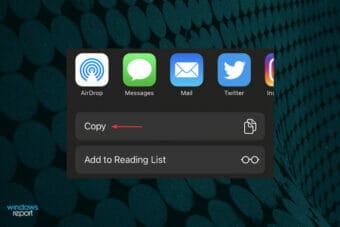This image captures a screenshot from a mobile app interface. The primary focus is a pattern of interconnected squares on a black background. These squares, displayed in a lighter gray color, intersect at non-right angles, forming an intricate design of triangles. Each triangle's interior is illuminated with a lighter shade, contrasting sharply against the dark background.

At the top of the image, there's a menu toolbar featuring several app icons. From left to right, the icons are:
- AirDrop, represented by a white square with concentric blue circles and a triangular cut-out.
- Messages, depicted as a green icon with a white speech bubble.
- Mail, shown as a blue icon with an envelope.
- Twitter, illustrated by a blue icon with a white bird.
- The edge of the Instagram icon is partially visible, suggesting its position at the far right of the toolbar.

Directly beneath this toolbar is the text "COPY," highlighted with a red arrow pointing towards it. Adjacent to this, on the right, is the copy symbol, depicted by two overlapping pieces of paper. Below this, the text "Add to Reading List" is visible, accompanied by an icon resembling a pair of glasses on the right side.

In the bottom left corner, there's some unreadable lettering, likely indicating the app's name. The entire layout of the image is rectangular, with the horizontal dimension being longer than the vertical.